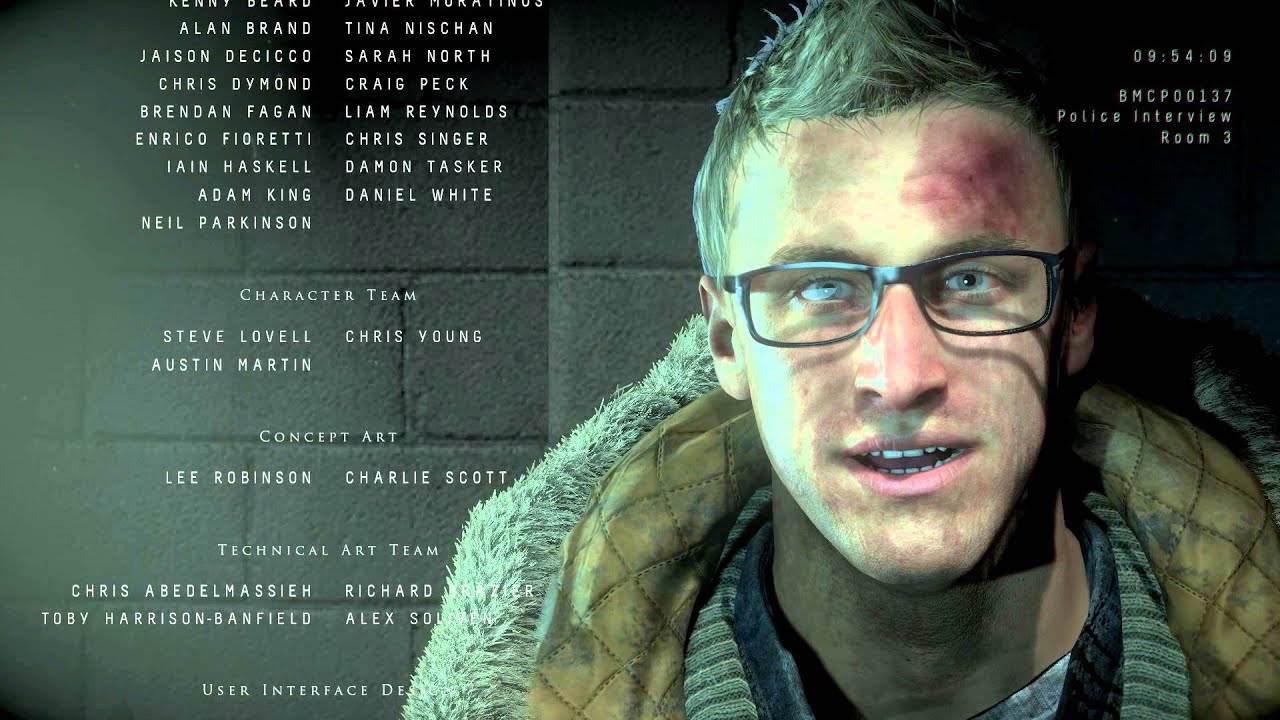The image depicts a man who appears to be in his 30s, standing against a background of black and gray cinder blocks. He looks somewhat disheveled and worse for wear, with a large bruise or red contusion on the top left side of his forehead and additional bruises on his face. His hair is messy, and he is wearing black glasses and a dirty green parka with fur around the hood over a sweater. The man's expression suggests a mix of emotions, possibly happiness or relief, despite his battered appearance. This scene is likely part of a media production, such as a movie or game, and resembles a police interview setting with the label "09-5409 BMCPOO137 Police Interview Room 3" on the right side of the image. On the left side, credits for the character team, concept art, technical art team, and character interface design are listed.